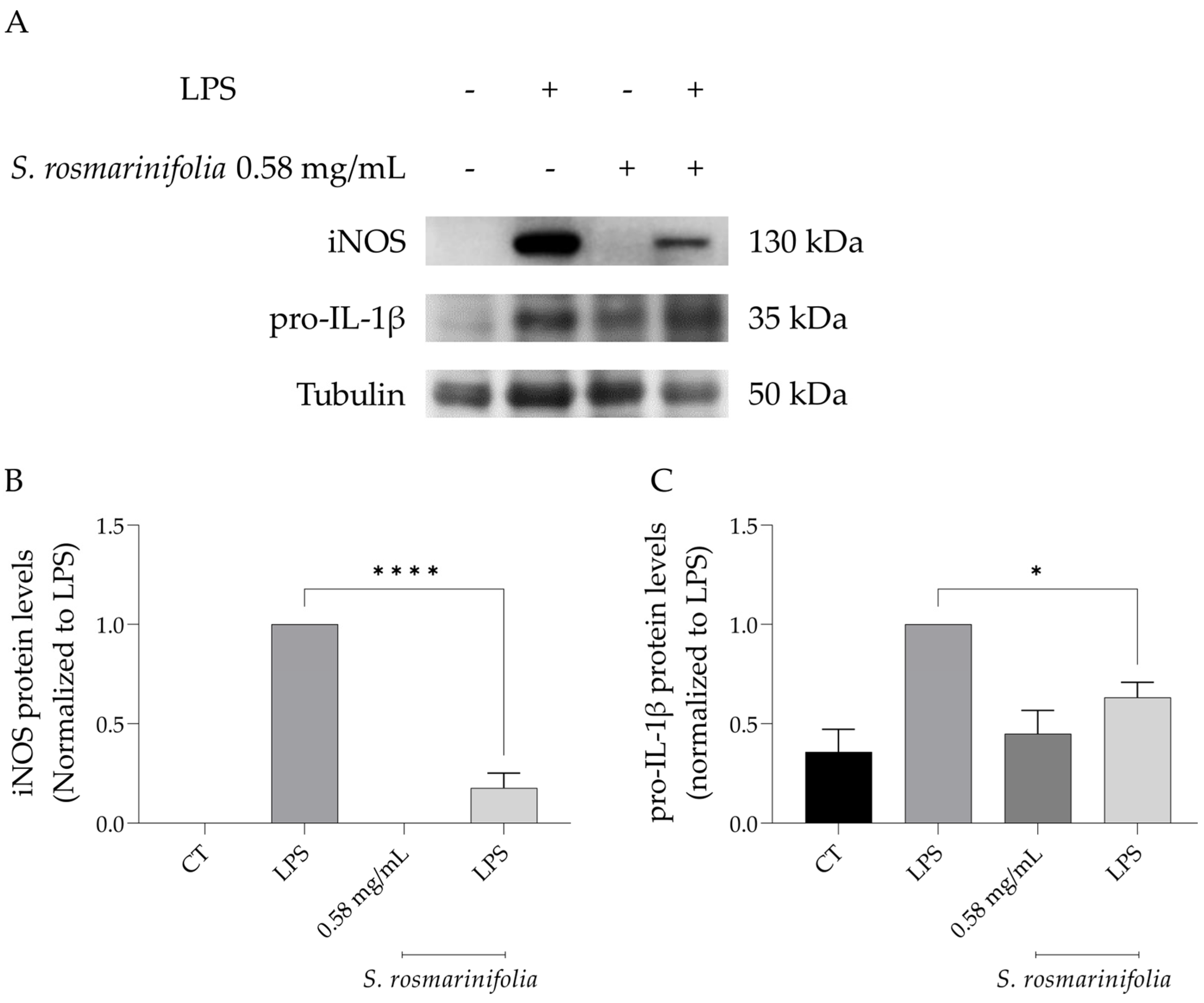The image consists of two sections: the top part displaying Western blot analyses and the bottom part featuring two bar graphs labeled B and C, respectively. 

The top section contains various chemical markers indicated by black and gray splotches against a white background. The labels in black text read "LPS," "S. rosmarinifolia," and "0.58 mg/mL." The specific components shown include "INOS," "130 kDa pro IL-1β," and "Tubulin," each with corresponding splotchy lines at different molecular weights: 130 kDa for pro IL-1β and 35 kDa presumably for Tubulin. There are also plus (+) and minus (-) signs associated with different experimental conditions.

The bottom section presents two bar graphs categorized under B and C. Graph B illustrates the "INOS protein levels normalized to LPS," while Graph C portrays "pro IL-1β protein levels normalized to LPS." Each bar within these graphs indicates varying protein levels, with vertical axes scaling from 0.0 to 1.5, marking distinct measured quantities.

Overall, this detailed depiction captures protein expression levels under the influence of LPS and S. rosmarinifolia, quantified and normalized in a structured, monochromatic layout.